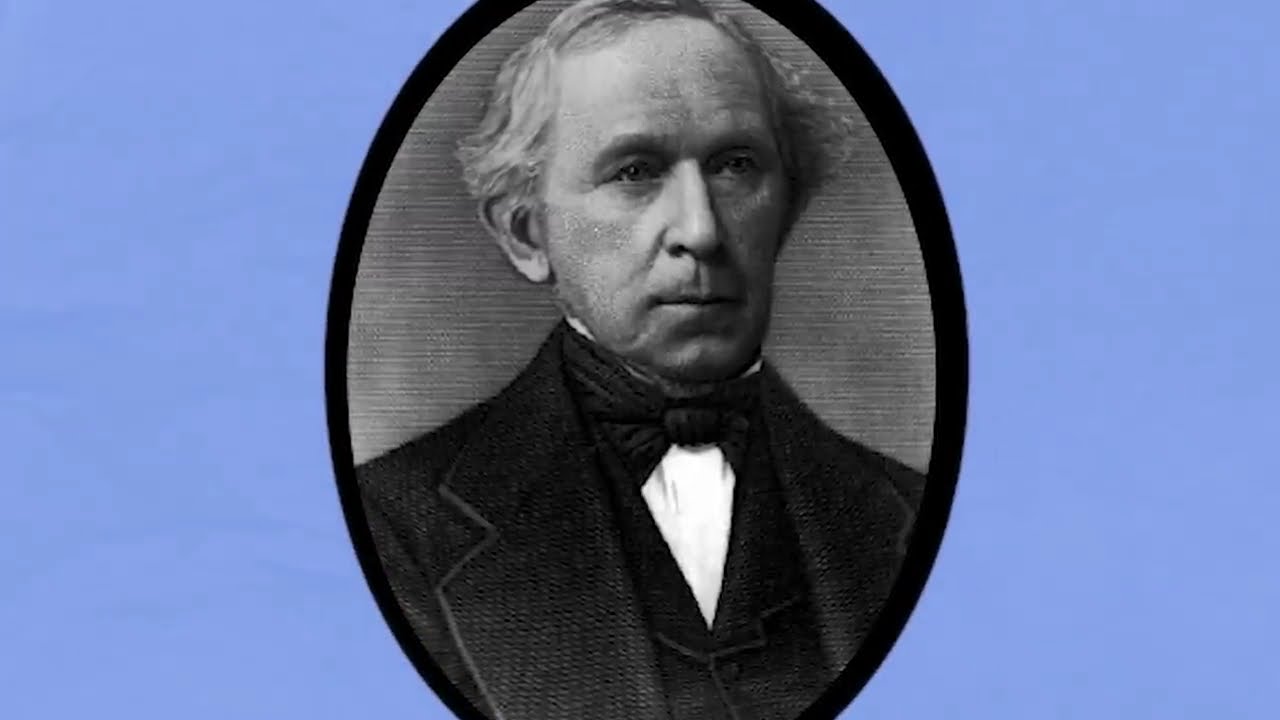The image depicts a black and white portrait of a man set against an elliptical, black background with an old-timey, vintage feel akin to a 19th-century photograph. The man, who appears to be Caucasian with light-colored, possibly gray hair parted on the right side, has a receding hairline with a lot of forehead showing. He is attired in formal, period clothing that includes a black suit jacket with wide lapels, a black waistcoat, a white shirt, and a distinctive bow tie resembling a large scarf tied around his neck. His stern face, lacking any facial hair, is oriented towards the viewer's right shoulder. Noteworthy is his visible, large left ear. The portrait, which conveys an official, almost presidential aura, is framed by a black oval with a lined, grainy texture, and set within a larger, rectangular slide that features a medium blue periwinkle background.